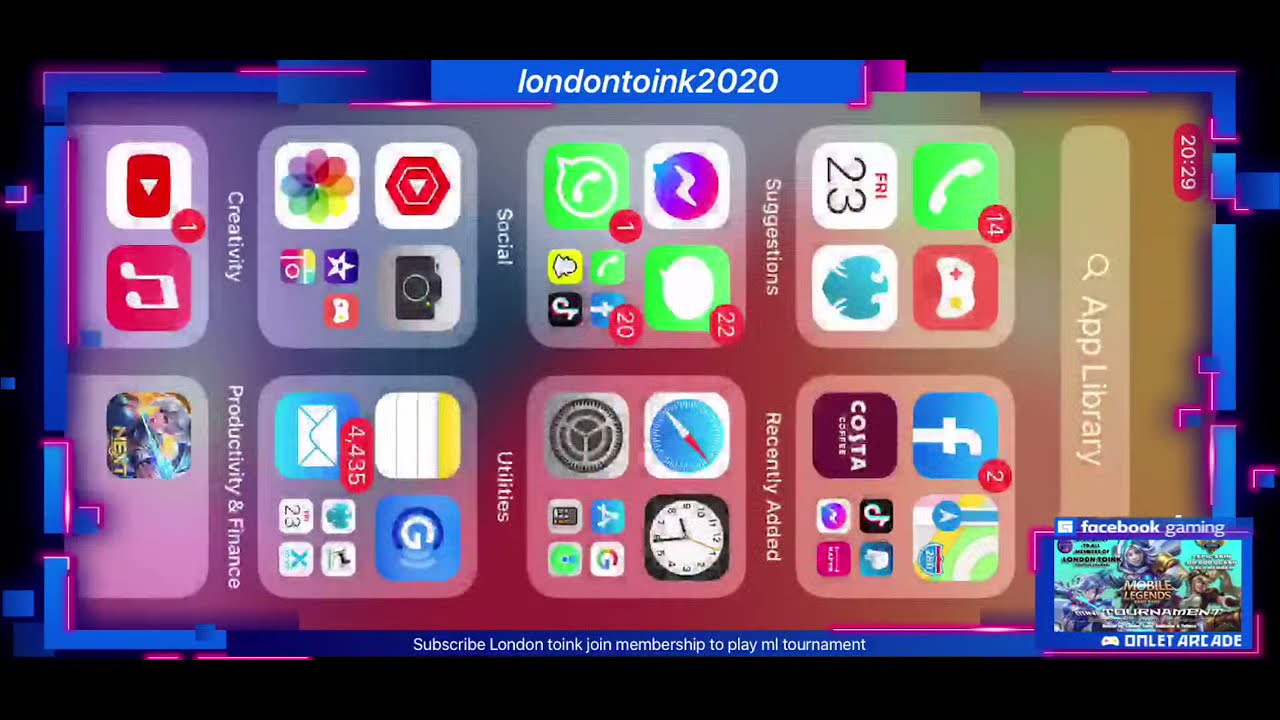The image is a detailed graphic screenshot of a cell phone's home screen, oriented horizontally with a black background. The phone screen is outlined in bright blue, creating a striking contrast. At the top center of the blue outline, it reads “London2Inc 2020” in white print. The bottom of the screen features the text “Subscribe London2Inc, Join Membership to Play MI Tournament.”

The main content shows the App Library of an Apple phone, illustrated with colorful icons grouped into various categories: Utilities, Social, Creativity, Productivity, and Finance. Specific app icons such as Clock, YouTube, Facebook, TikTok, Snapchat, and Google apps are visible, alongside a screen recording app, Compass, Phone dialer, and a Music app. The day is marked as Friday the 23rd.

In the lower right corner, there’s an area labeled “Facebook Gaming Onlit Arcade,” and just above it with a red background, the number “2029” is displayed prominently. Various other app groups are visible, including clusters for gaming, calendar, maps, Messenger, camera, images, notes, and emails. The overall layout suggests the screen has been laid on its side, requiring viewers to tilt their heads to read conveniently.